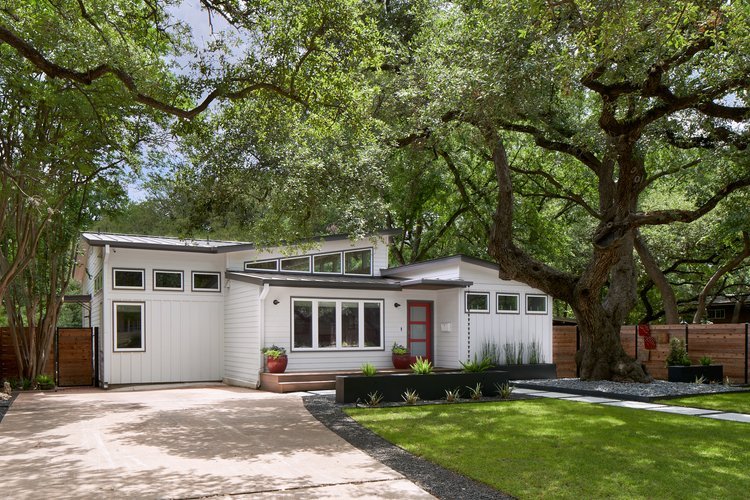This outdoor photograph depicts a tastefully remodeled single-story house with white siding and gray trim, combining modern and traditional elements. The roof is gray and features a unique, angular design with various triangular windows. Prominently, the house has a red wooden door with three glass panes, framed by white-bordered windows. The neat front lawn showcases both green grass and desert plants, alongside strategically placed rocks and planters. A large tree, encircled by gravel, stands to the right, accompanied by a smaller tree on the left. The property is framed by a wooden fence on both sides, and the concrete driveway lies to the left, while a concrete walkway resides on the right, leading to a small, tidy porch with potted plants. This sunlit image, likely taken from a real estate listing, exudes a serene, lush summer atmosphere amidst a tree-filled background.